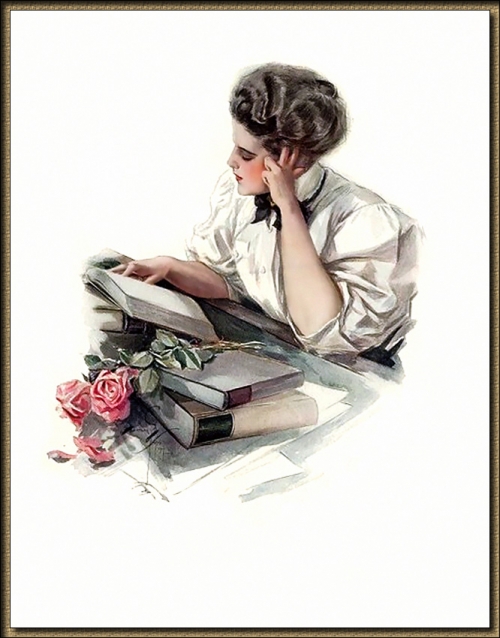The image is a painting depicting a contemplative woman in her 30s or 40s, with coiffed hair styled in an elegant up-do and wearing makeup. She is captured in profile from the left, with her head resting thoughtfully on her left hand, her pointer and middle fingers extended along her cheek. Dressed in a white blouse featuring elbow-length, flounced puffed sleeves, she has a white neckerchief or necktie tied in a bow around her neck. She is seated at a grey table, engrossed in reading a book she holds open with her right hand. In front of her, two additional light brown books are stacked, adorned with two pink roses, complete with leaves. The background and the edges of the painting are entirely white, framed by a very thin brown border. The composition focuses solely on the woman and her reading, emphasizing an atmosphere of quiet contemplation and concentration.